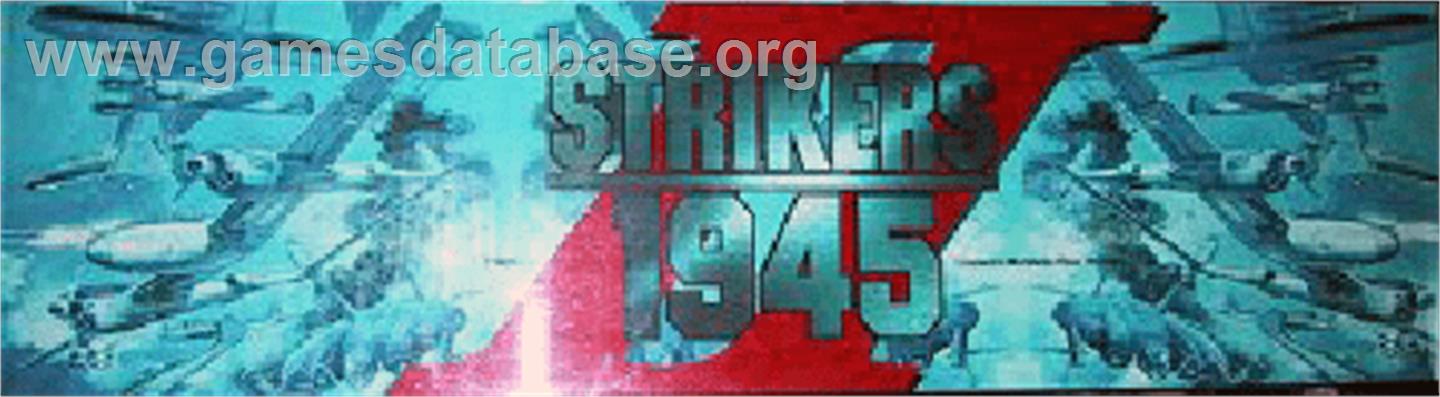The image showcases a promotional banner for a computer game called "Strikers 1945," which appears to be themed around World War II aerial combat. The background predominantly features various shades of blue, interspersed with white, red, brown, and gray. At the top left corner of the banner, the text "www.gamesdatabase.org" is displayed. Centrally positioned in large gray lettering is the game's title, "Strikers 1945," emphasized by a red backdrop. To the left of the title, several low-resolution graphical representations of military aircraft, including bombers reminiscent of World War II-era planes, are depicted flying through the sky. Additional aircraft are visible scattered throughout the banner, reinforcing the theme of air-based warfare and supporting the retro, early video game stylization of the entire image.